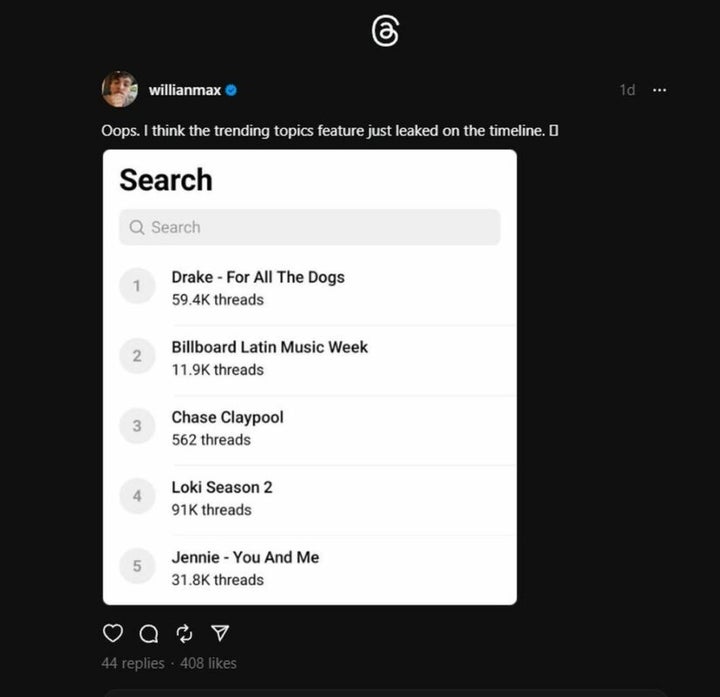This vertical, black background image, seemingly from a social media platform like Twitter, is a composition rich in detail. The solid black background serves as a stark contrast to the contents within the frame, providing a one-dimensional, flat canvas.

At the top of the image, there is an intricate, swirly white design resembling a stylized sea, with a distinctive font featuring the letter "A" embedded within it. Below this, on the left side, appears a circular profile picture of a user named "William Max," accompanied by a blue circle with a black checkmark, indicating a verified account. To the right of the profile picture, the text "one day..." is displayed, suggesting the tweet was posted a day ago.

Beneath William Max's name is his tweet which reads: "Oops, I think the trending topics feature just leaked on the timeline." This tweet is followed by a white vertical box prominently displaying the word “Search” in bold black letters. Below the search bar, five trending topics are listed, each within a gray circle representing numerical ranking and trending content:
1. "Drake for all the dogs" with 59.4k threads,
2. "Billboard Latin Music Week" with 11.9k threads,
3. "Chase Claypool" with 562 threads,
4. "Loki season 2" with 91k threads,
5. "Jenny, you and me" with 31.8k threads.

At the bottom of the image, there are interactive icons commonly found on social media: a heart symbol, a chat bubble, a share arrow, and a paper airplane icon. Accompanying these icons are statistics indicating user engagement: 44 replies and 408 likes.